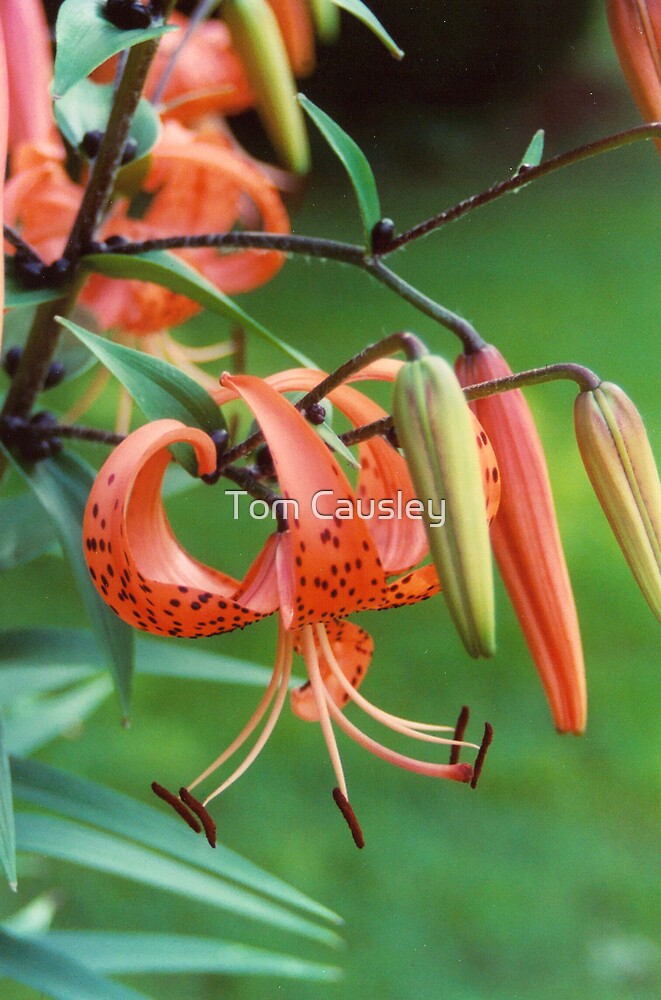In the photograph, the central focus is on a striking orange flower with distinctive black spots on its elongated petals, which gracefully curl backward. Emerging from the heart of the flower are prominent, long tendrils that culminate in brown-tipped structures, likely where pollination occurs. The vivid blossom resides on a branch adorned with a mix of green leaves and several unopened buds, hinting at various stages of bloom. The background is a soft, blurry green, creating an outdoor ambiance and featuring glimpses of slender, palm-like leaves, though they are not from a palm tree. This blurred greenery accentuates the detailed clarity of the central flower and its accompanying elements, underscoring the natural beauty and intricate details of the plant.